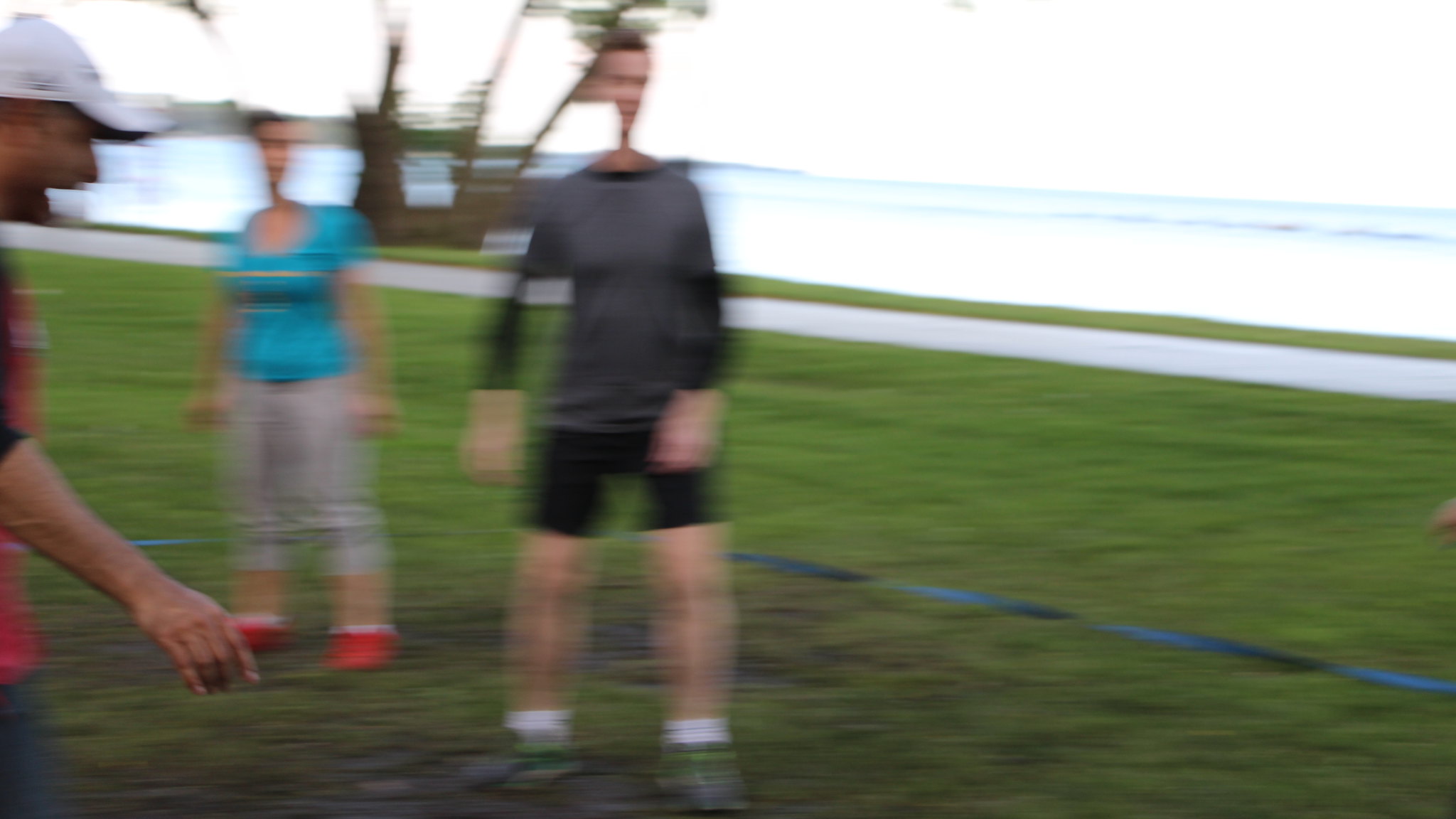In this blurry image, three individuals are standing in a grassy field. The first person, on the left, is dressed in a dark long-sleeved shirt paired with dark-colored shorts, white socks, and gray shoes. The second person, in the center, is sporting a blue tank top with a yellow section on the front, gray sweatpants, and red-and-white shoes. The third individual, mostly cropped out of the frame on the right, is wearing a white hat and a red top with dark-colored sleeves. The vibrant green grass underfoot is interrupted by a blue gradient line running along the ground. In the background, a stone pathway leads to what appears to be a body of water with visible waves, set against a gray sky.